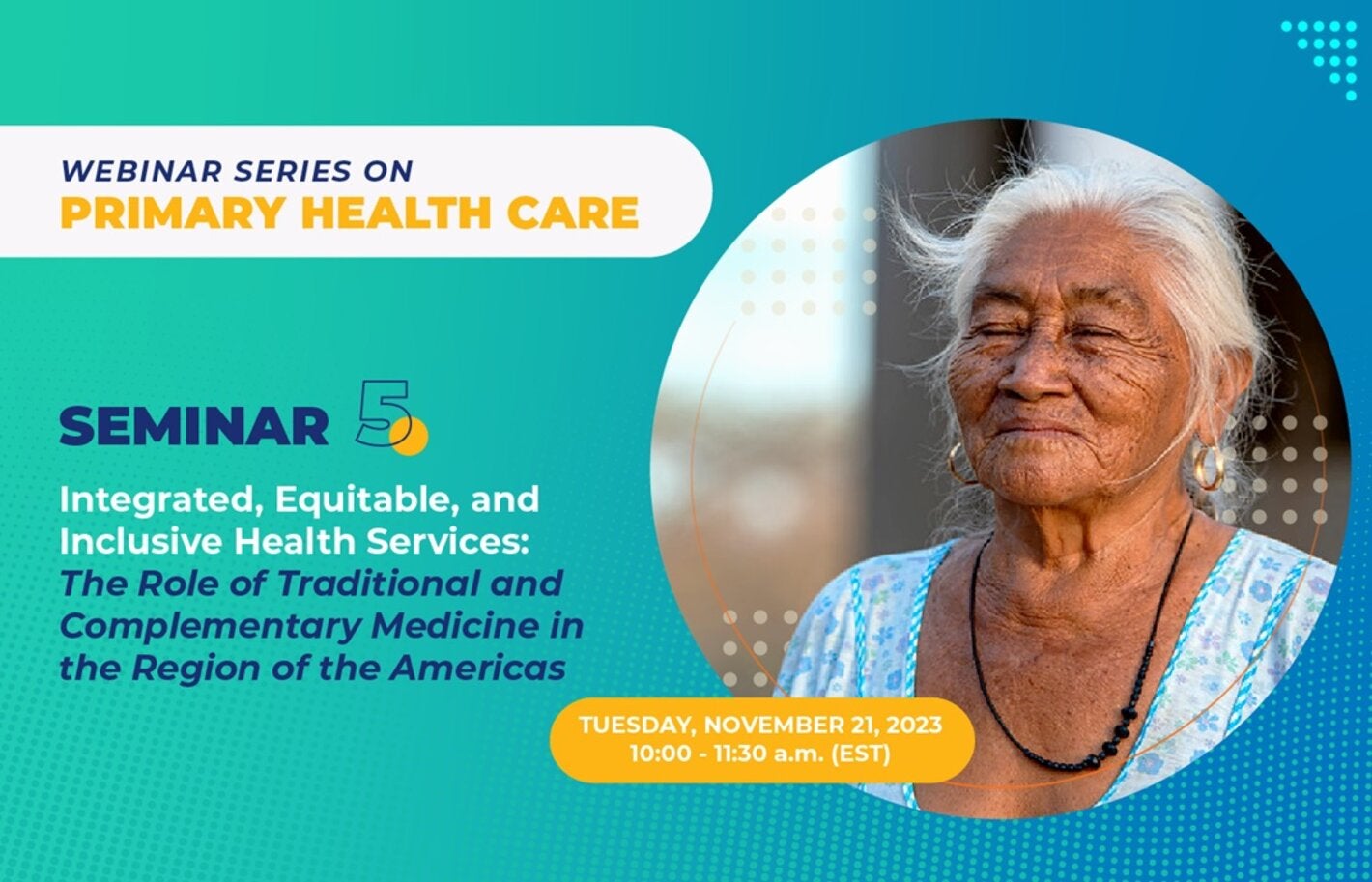The advertisement for a webinar series on primary health care features a serene image of an elderly, possibly Native American woman with dark skin and completely gray-white hair. She is smiling blissfully with her eyes closed, adorned with white hoop earrings, a black necklace, and a blue dress. The background transitions from a light lime green on the left to a light blue on the right, with various dotted patterns: light blue dots forming a triangle in the upper right corner, light green dots in the lower right, and light blue dots in the lower left. The top left corner bears the text in white: "Webinar Series on Primary Health Care." Below it, additional details about the event include: "Seminar 5 – Integrated, Equitable, and Inclusive Health Care Services, the role of traditional and complementary medicine in the region of the Americas." The event is scheduled for Tuesday, November 21, 2023, from 10:00 to 11:30 a.m. Eastern Standard Time, indicated in a prominent yellow circle.